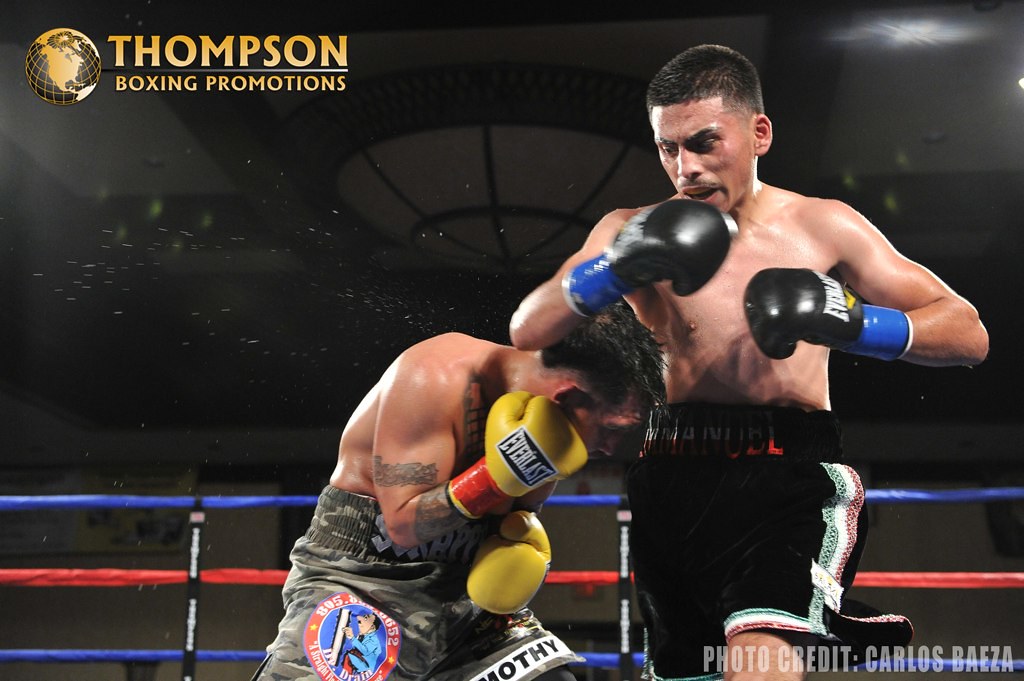The image shows an intense moment in a boxing ring featuring two fighters under the bright lights of an auditorium with blue and red ropes visible in the background. The boxer on the right, dressed in black trunks with green, white, and red stripes, has short black hair and a short mustache. He stands poised to strike with black Everlast gloves that feature blue wraps around the wrists. Opposite him, the boxer on the left, wearing camouflage trunks, is ducking under his opponent's punch while protecting himself with yellow Everlast gloves that have red wraps. This fighter has noticeable tattoos on his right bicep and forearm. The environment around the ring is dark, obscuring any audience, placing full attention on the action in the ring. Above, the image includes promotional graphics for Thompson Boxing Promotions, featuring a globe highlighting the United States and a checkered pattern, with the logo text in a yellow-to-white gradient. In the lower right corner, the photo is credited to Carlo Beza.